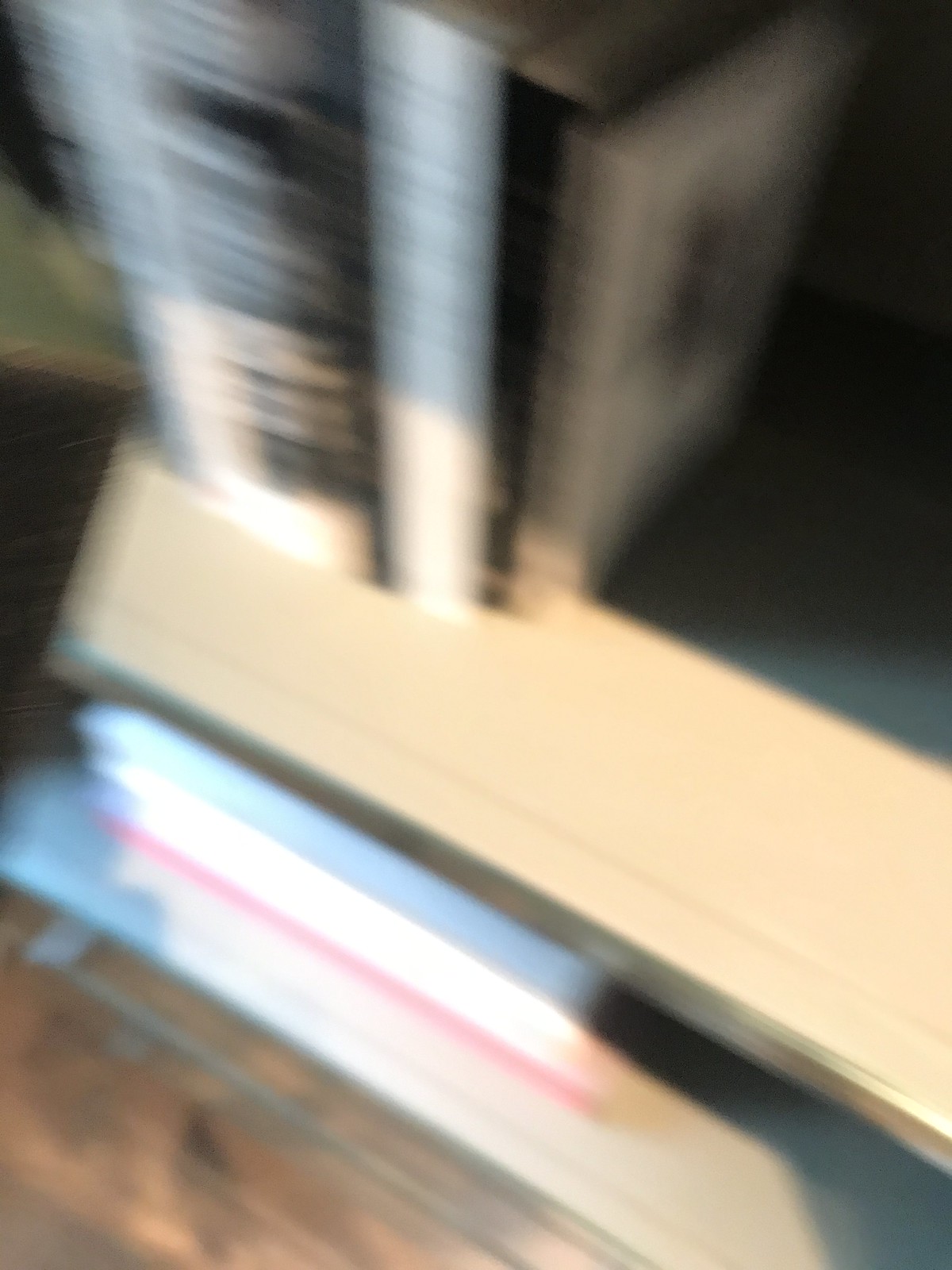This photograph, though very blurry and lacking clear detail, depicts a scene likely involving a bookshelf viewed from above. At the top of the image, there are at least three or four books of various widths, one of which is quite wide and positioned on the left side. Three narrower books are to its right, their spines gray and partially illuminated by sunlight. To the right of these books is a gray, shaded area. The bookshelf appears to be made of light brown wood, and is illuminated by sunlight falling on its surface.

Beneath this wooden shelf is another shelf made of glass. On this glass shelf, there are a couple of books or magazines placed horizontally, including some white paper with a blue top and possibly a pinkish bottom. The lower left-hand corner of the image shows a section of a wooden floor. Despite the image's graininess and blur, it is clear that there are no visible people or living things, nor any readable text on the book spines or covers. The overall impression is of a well-lit, possibly sunlit, domestic interior, with a focus on the arrangement and placement of books on a wooden and glass shelving unit.